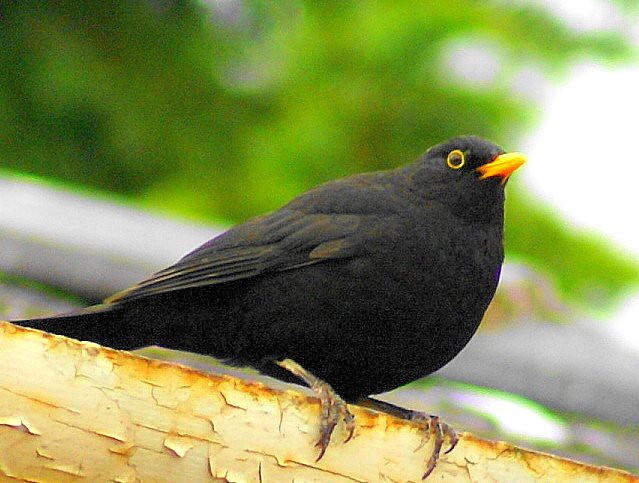This photograph, taken in bright daylight, captures a small but chubby black bird perched on a piece of aged, chipped yellow-painted wood that stretches diagonally across the image from the bottom left to the bottom right corner. The bird is centered toward the bottom of the frame, facing slightly forward and to the right. Its glossy black feathers are in sharp focus, contrasting with its striking orange beak and a distinctive yellow rim around its eye. The bird's skinny legs and long claws are firmly gripping the wood, which is cracked and peeling, suggesting it was once painted. The background is a blurry mix of green hues, likely indicating distant trees or foliage, adding depth while keeping the focus squarely on the bird.